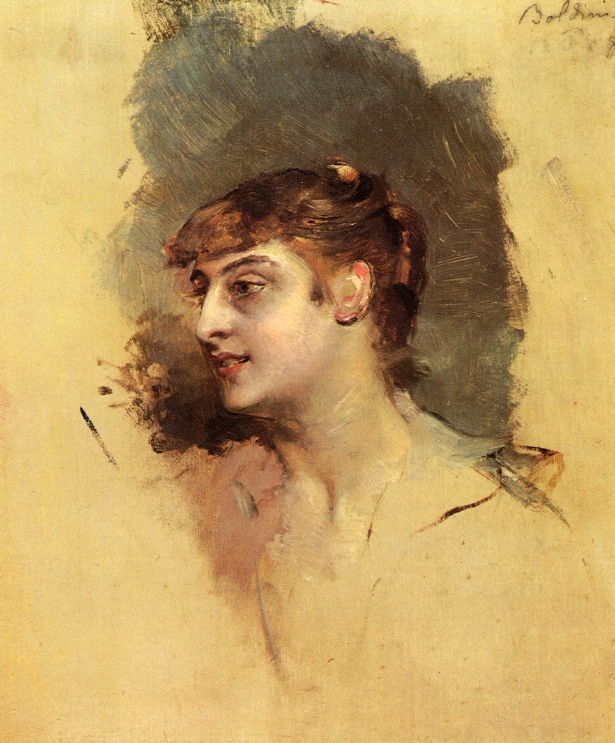This is an unfinished portrait of a woman with European features, captured in a side profile with her gaze directed to the left. The painting reveals her from the neckline upwards. She has amber-brown hair that is tightly braided and pulled back, with a touch of bangs framing her face. Her complexion has a distinct gray tint, blended with peach tones, especially prominent on her nose and the side of her head. Her face displays highlighted cheekbones, strong eyebrows, and detailed eyes surrounded by subtle makeup. 

The artist has given her an inquisitive smile, with her lips slightly parted, revealing a glimpse of her teeth; her lips are painted in a soft orange-red hue. There's a small pink smudge within her ear and a noticeable dark brown spot underneath the earlobe. The background transitions around her head from dark brown to smoky gray and expands into a yellowish hue beyond, matching the area around her subtly portrayed shoulder. The overall canvas carries an intentionally unfinished quality, with parts of her collar and shoulder merely outlined and fading away, lending a deliberately unrefined and aged appearance, reminiscent of 18th to 19th-century portrait styles.